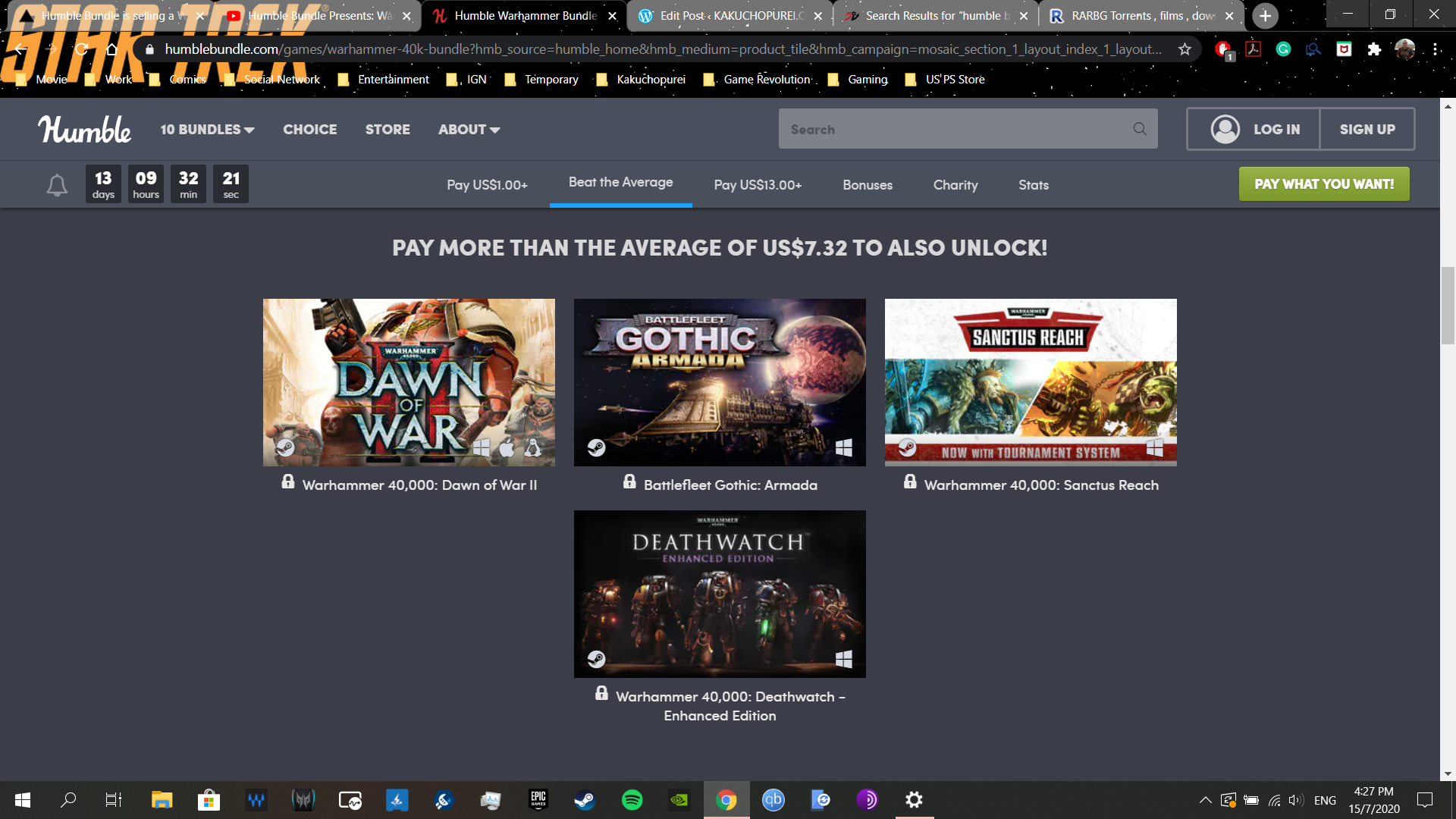This image is a detailed view of a webpage from the Humble Bundle website, specifically showcasing a Star Trek-themed promotion. At the top of the page, the browser tabs display "Humble Bundle presents W" alongside "Star Trek." The brand's logo "Humble" is written in cursive. Below the logo, the site navigation includes tabs labeled "10 Bundles," "Choice," "Store," and "About." A search bar, login button, and sign-up button are also visible, followed by a notification bell.

Below these elements, a series of countdown timers are displayed in black squares, counting down 13 days, 9 hours, 32 minutes, and 21 seconds. Following this, pricing options are listed: "Pay US$1.00+," "Beat the Average, Pay US$13.00+," and additional options for "Bonuses," "Charity," and "Stats." A prominent green call-to-action button urges users to "Pay What You Want."

The main content features visuals of various Warhammer 40,000 games available in the bundle. The first image depicts "Warhammer 40,000: Dawn of War II," showcasing a warrior in red and gold armor holding a machine gun with the game's title written in blue. Next is "Battlefleet Gothic: Armada," illustrated with a spacecraft and planet. Another game, "Warhammer 40,000: Sanctus Reach," features a blue monster facing a gold monster with a slash dividing them, highlighting the new tournament system. Finally, "Warhammer 40,000: Deathwatch Enhanced Edition" shows a group of warriors or creatures.

At the bottom of the screen, a series of application icons are visible, indicating various other functionalities available from the Humble Bundle website.